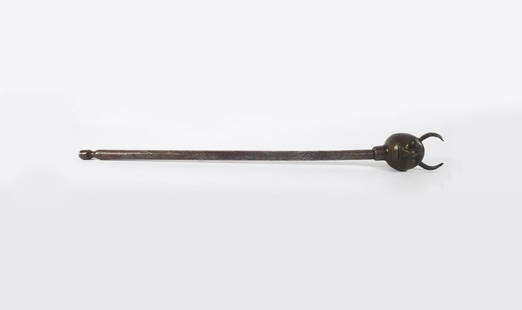The photograph features a small, cylindrical metal device on a white, semi-reflective background. The object is predominantly black with a noticeable transition from silver at the left end to black at the right end. The left side resembles a drill bit, suggesting it might be inserted into a drill. The right side culminates in a spherical head with two horn-like fangs protruding from it. The spherical head has two dents on its surface, possibly indicating a face-like design. The overall appearance, including the shiny but dull reflective surface, suggests it could be made of either metal or semi-rigid plastic. The intriguing design hints at it being a specialized tool or a decorative handle, like that of a cane or walking stick.